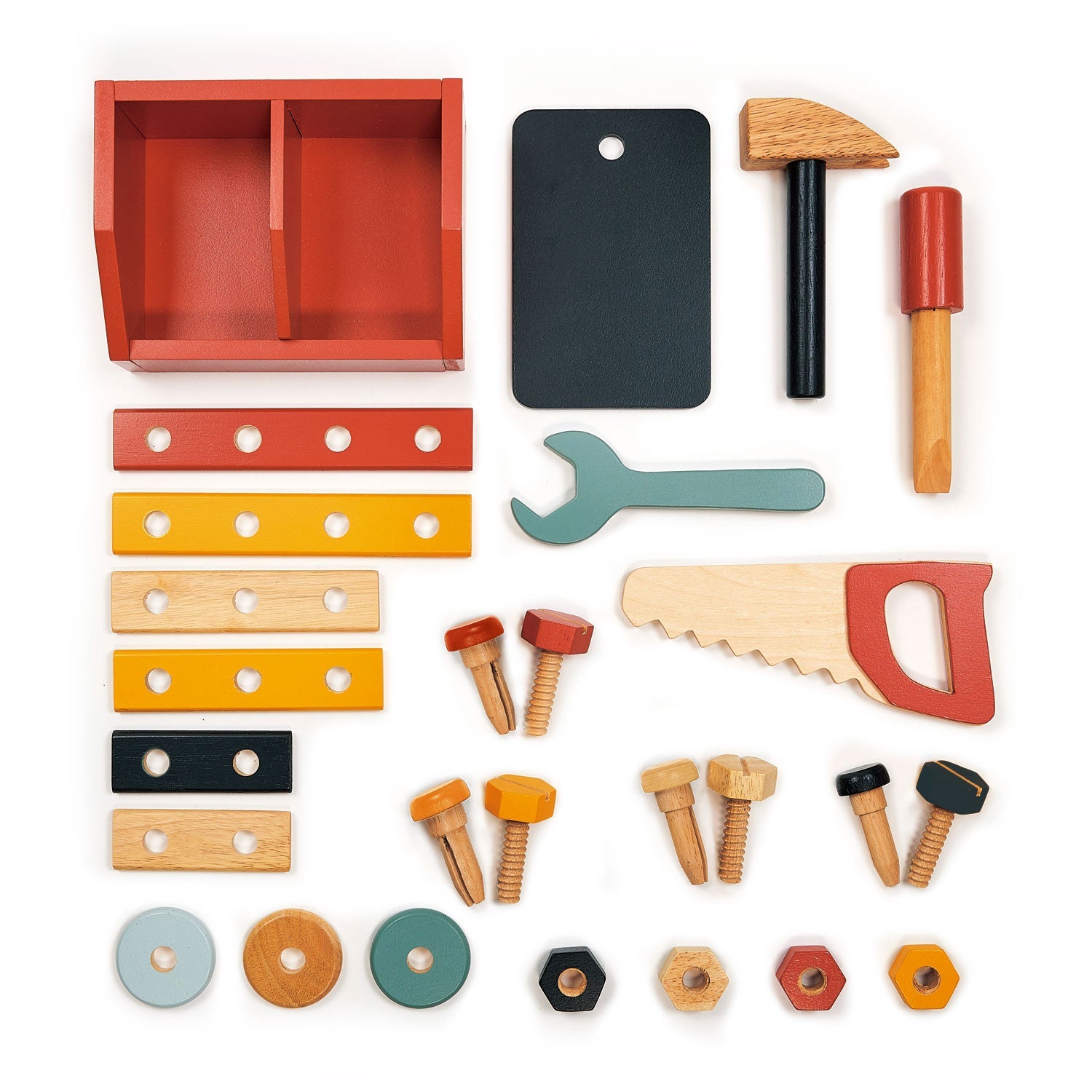The image depicts a vibrant, multicolored children's toy tool set, meticulously laid out without a border or background. This set, likely made from wood or plastic, includes various toy tools such as a hammer, a screwdriver, a wrench, and a small saw. Scattered among these are several screws, nuts, bolts, and washers, as well as colored strips with holes for inserting screws. The tools cast subtle shadows, and the scene is predominantly colored in reds, yellows, and blues, creating an engaging and playful atmosphere. This set allows children to mimic construction activities safely and imaginatively, offering them the fun experience of building and fixing things.